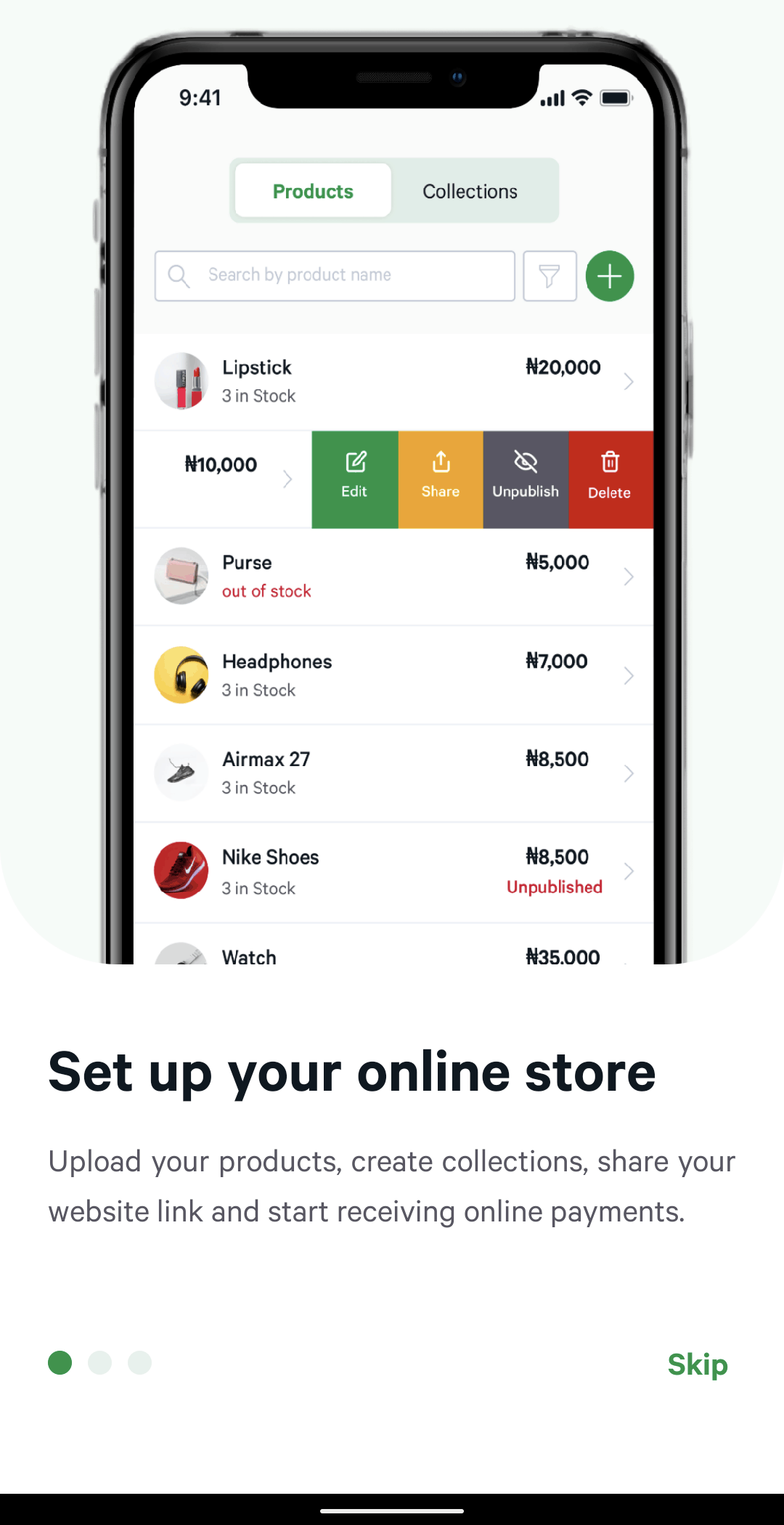The image showcases a smartphone displaying a user interface for managing an online store. At the top, there are two tabs: "Product" (highlighted in green) and "Connections" (in black). Directly beneath the tabs is a search bar prompting users to "search products by name," flanked on the right by a filter icon and a green circular add button with a white plus sign.

The main content lists various products:

1. **Lipstick**: In stock (3), priced at 20,000 Naira. Below the product name are four action buttons: "Edit" (green), "Share" (orange), "Publish" (grey), and "Delete" (red).
2. **Unnamed Second Product**: Costs 10,000 Naira (not shown in detail).
3. **Pants**: Out of stock, priced at 5,000 Naira.
4. **Headphones**: In stock (3), priced at 7,000 Naira.
5. **MX27**: In stock (3), priced at 8,500 Naira.
6. **Nike Shoes**: In stock (3), priced at 8,500 Naira, marked as unpublished with a red "unpublished" label.
7. **Watch**: Priced at 35,000 Naira.

Beneath the displayed products, outside the main user interface, there is a white background with black text, providing instructions: "Set up your online store, upload your product, create connections, share with your website link, and start receiving online payment." At the bottom right corner, a green "Skip" button is visible, indicating that this tutorial or setup guide can be skipped.